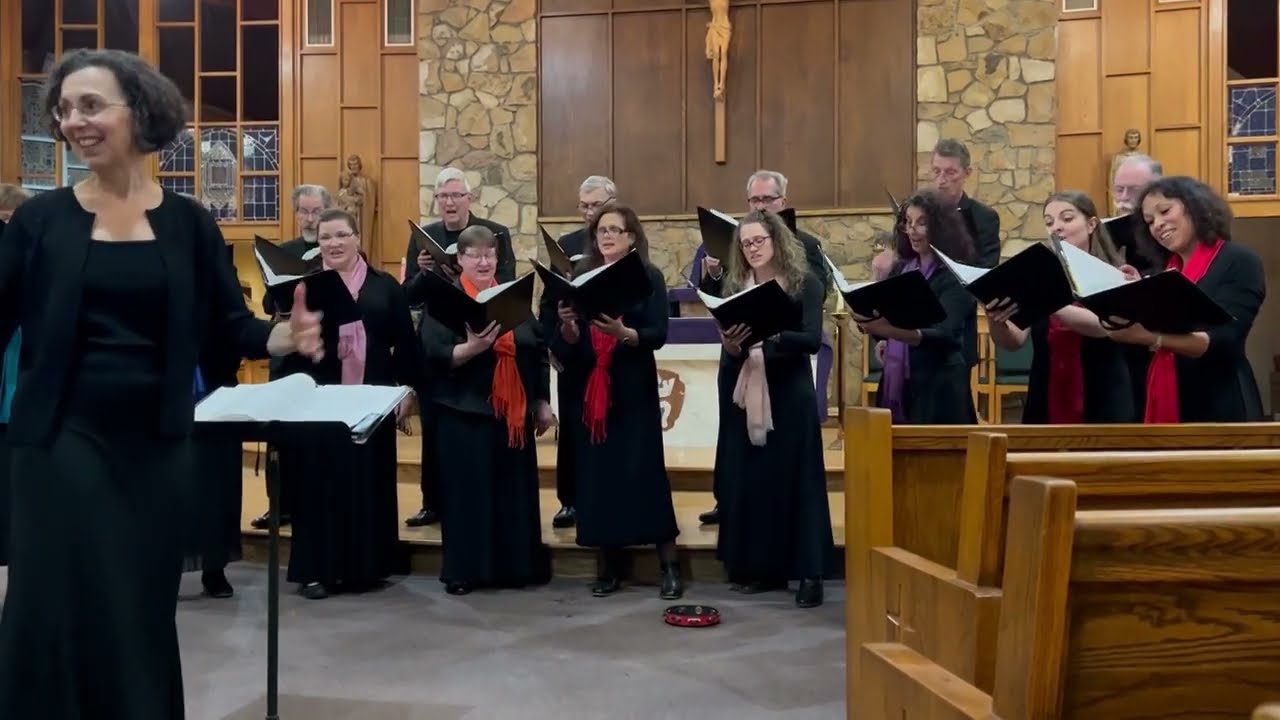The image captures a vividly detailed scene of a church choir performance in a traditional chapel setting, presented in a landscape-oriented color photograph. Approximately 14 individuals, a mix of men and women, are adorned in black robes and colorful sashes in hues such as purple, pink, red, and blue. They are singing from black binders, exuding joy and engagement. The choir stands on a light cement floor, with a stage and partial church pews visible on the right. The chapel features large stone walls with wooden paneling surrounding a partially visible statue of Christ on the cross, creating a serene backdrop. Large windows flank the scene, revealing the night outside. Dominating the foreground on the left, a smiling woman in a long black dress and sweater is directing the choir, her black music stand holding white sheet music. The overall style of the photograph emphasizes realistic and representational details.